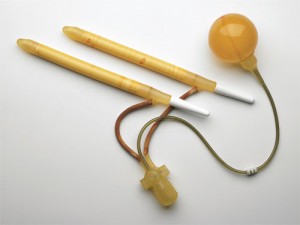The photograph showcases a mechanical device against a white background that transitions to light gray at the bottom. Central to the image are two elongated, cylindrical elements resembling retractable chopsticks, which are angled slightly diagonally from the upper left to the middle center right. These "chopsticks" have light bamboo-colored wooden handles, capped with retracted white nubs on one end. They are interconnected via a network of wires or tubes with an aging, yellowed plastic connector that splits into two red wires, each connecting to one of the cylindrical elements. Another green wire extends from this connector to a separate bulbous object, somewhat resembling a golf ball, situated in the upper right corner. This object also appears to be made of yellowed plastic, suggesting it may have once been clear. Additionally, the cylindrical elements are lying on what seems to be a leather or hemp lanyard, equipped with small mustard-yellow caps or closures, possibly for securing the cylinders together when not in use. Overall, the device appears to involve components that suggest functionality for pumping air or heating, enveloped in a web of aging plastic and colored wires.